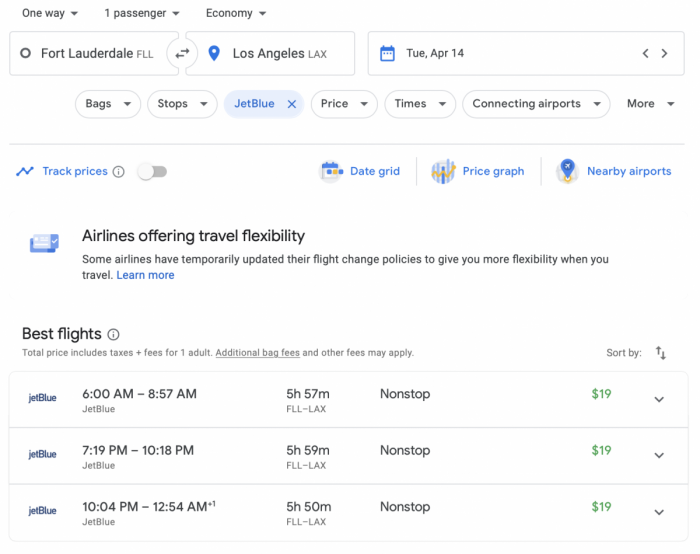**Detailed Descriptive Caption:**

The image is set against a crisp white background, showcasing a flight search interface. At the top left, the text is displayed in black font, starting with options for "One Way" accompanied by a small downward triangle, "One Passenger" with a pull-down menu, and "Economy" with another pull-down menu.

Below these options, the interface presents a series of fields. The first horizontal field features "Fort Lauderdale" with the airport code "FLL" next to it. Adjacent to this, a circular icon with arrows indicates a round-trip toggle. To the right, there’s a blue teardrop-shaped icon next to "Los Angeles" with the airport code "LAX."

The subsequent field is dedicated to the travel date, featuring a blue calendar icon to the left, followed by "TUE, APR 14."

Underneath this, there are several pull-down menu options displayed within horizontal ovals, each marked by a small downward triangle. These are labeled "Bags," "Stops," and in light blue, "JetBlue" with an "X" on the right side. The next options revert to black for "Price," "Times," "Connecting Airports," and finally, "More," which is not enclosed in an oval but remains aligned with the others.

A faint light gray line divides this section from the next, where, to the left, there is a "Track Prices" option in blue, complete with an accompanying icon and an off-position toggle switch.

In the middle and extending to the right, there are tabs in blue that read "Date Grid," "Price Graph," and "Nearby Airports," separated by fine gray lines and each with a corresponding logo to the left.

Below this section, a notification titled "Airlines Offering Travel Flexibility" appears, along with an icon. The text explains that some airlines have temporarily updated their flight change policies for enhanced travel flexibility, followed by a "Learn More" link in blue.

The "Best Flights" header is displayed in black, and beneath it, a disclaimer notes that the "Total price includes taxes and fees for one adult," with a reminder that additional bag fees and other charges may apply.

Finally, the image lists three flight options from JetBlue. Each listing includes the departure and arrival times, the flight duration, and the route code "FLL-LAX." All flights are marked as nonstop and are highlighted in green with a price of "$19."